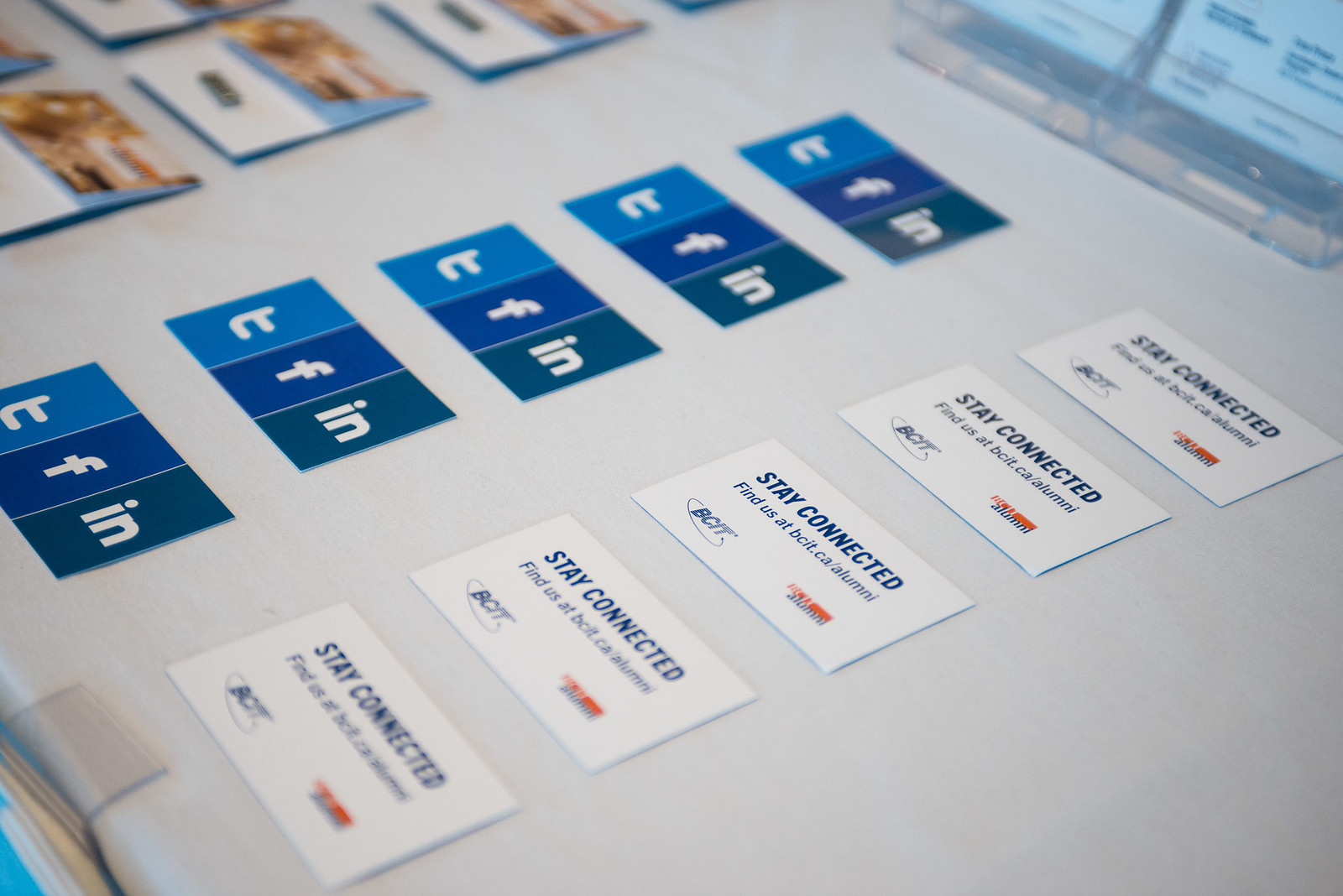In the image, a white table serves as the base for an arrangement of various cards and labels, suggesting a setting like a job fair or conference. On the left-hand side of the table, there's a vertical row of three distinct cards: a light blue card featuring a 'T' for Twitter, a dark blue card with an 'F' for Facebook, and a green card displaying 'IN' in white font for Indeed. Adjacent to this row, to the right, lies a white business card that reads "Stay connected" in bold black letters, followed by the URL "find us at bcit.ca/alumni." Below this phrase is the BCIT logo, with an additional red and blue logo whose details are unclear. Further right, and slightly above, the table holds five light blue cards and two dark blue cards running down its middle, which contain partially obscured text that seems to say 't-f-n.' The left-upper corner and lower-left side of the picture feature more blue-tinted, blurred labels, while the upper-right corner appears to have some sort of screen or electronic display, potentially a laptop or an iPad, contributing to the professional ambiance of the scene.